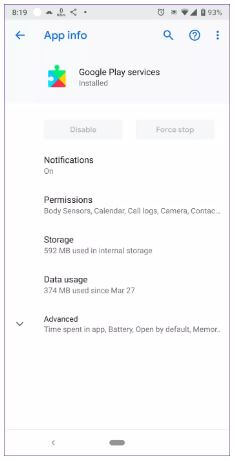The screenshot taken from an Android cell phone displays detailed information from the 'App Info' page of the Google Play Services app. The time on the phone reads 8:19, and the battery charge is at 93%. Various icons are scattered across the status bar at the top. 

The navigation bar at the top of the 'App Info' page features a blue arrow pointing left to go back, the words "App Info" in blue, and three icons on the right: a magnifying glass for search, a question mark inside a circle for help, and three vertically aligned dots for additional options.

The main section highlights the Google Play Services app, with its status marked as "Installed" next to a puzzle piece icon in Google's signature colors: blue, red, yellow, and green. Below the app's name are two grayed-out buttons labeled "Disable" and "Force Stop," indicating they are not selectable.

Further down, the word "Notifications" is bolded, with "On" underneath, indicating notifications for the app are enabled. The next section, titled "Permissions," lists the app's granted permissions: body sensors, calendar, call logs, camera, and contacts.

Following this, the "Storage" section is bolded, showing that 592 MB of internal storage is used. The "Data Usage" section notes that 374 MB have been used since March 27th. An "Advanced" section is also bolded, with sub-sections including "Time spent in app," "Battery," "Open by default," and a partially visible text beginning with "MEMOR...", indicating possibly 'Memory'. To the left of the "Advanced" label, an arrow suggests an expandable menu, though it is currently collapsed, concealing further details.